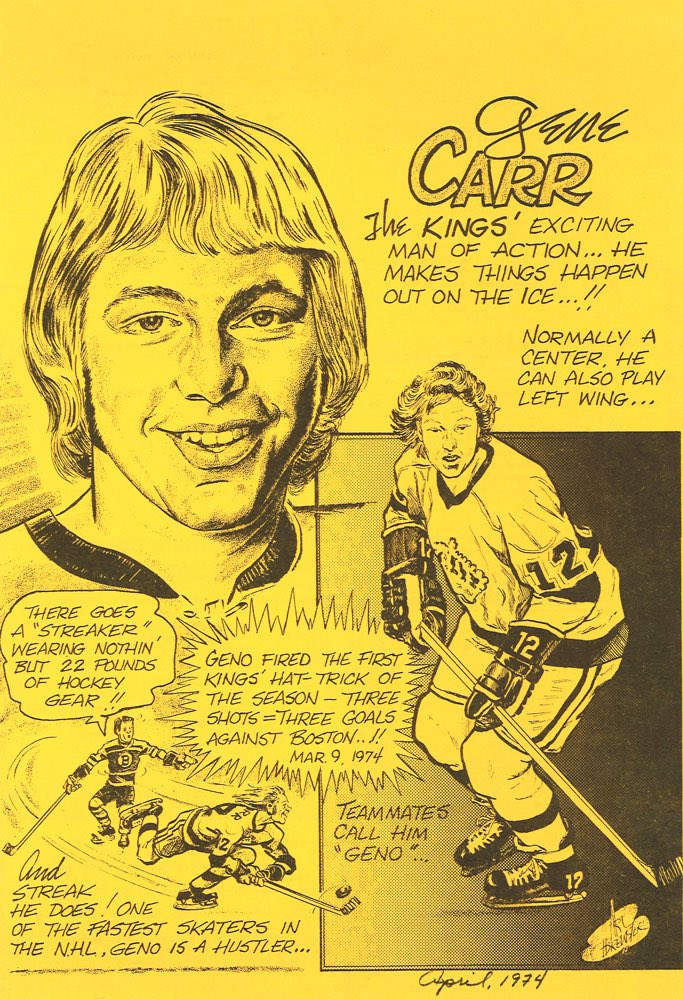The image, reminiscent of a comic or a magazine clipping from April 1974, showcases Gene Carr, a standout player for the Kings known for his versatility and dynamism on the ice. Predominantly yellow, the background features several black sketches of Carr, each reinforcing his reputation as a powerhouse in hockey. The largest depiction is a close-up of his face with a bowl-shaped haircut, giving his head a square look, and a welcoming smile. Below this, another sketch presents Carr in full hockey gear, speeding across the ice with a puck, highlighting his agility and speed.

Further down, additional full-body sketches emphasize Carr's physicality and his hustle, capturing him mid-action. Prominent text across the image notes his nickname, "Geno," and celebrates his impactful performances, such as his first hat trick of the season against Boston on March 9, 1974. Another playful quote reads, "There goes a streaker wearing nothing but 22 pounds of hockey gear," underlining his light-hearted persona. The entire composition, consisting of hand-drawn illustrations and handwritten captions, captures the essence of an exciting, multifaceted athlete who is as versatile as he is fast, often switching between center and left wing positions for the Kings.